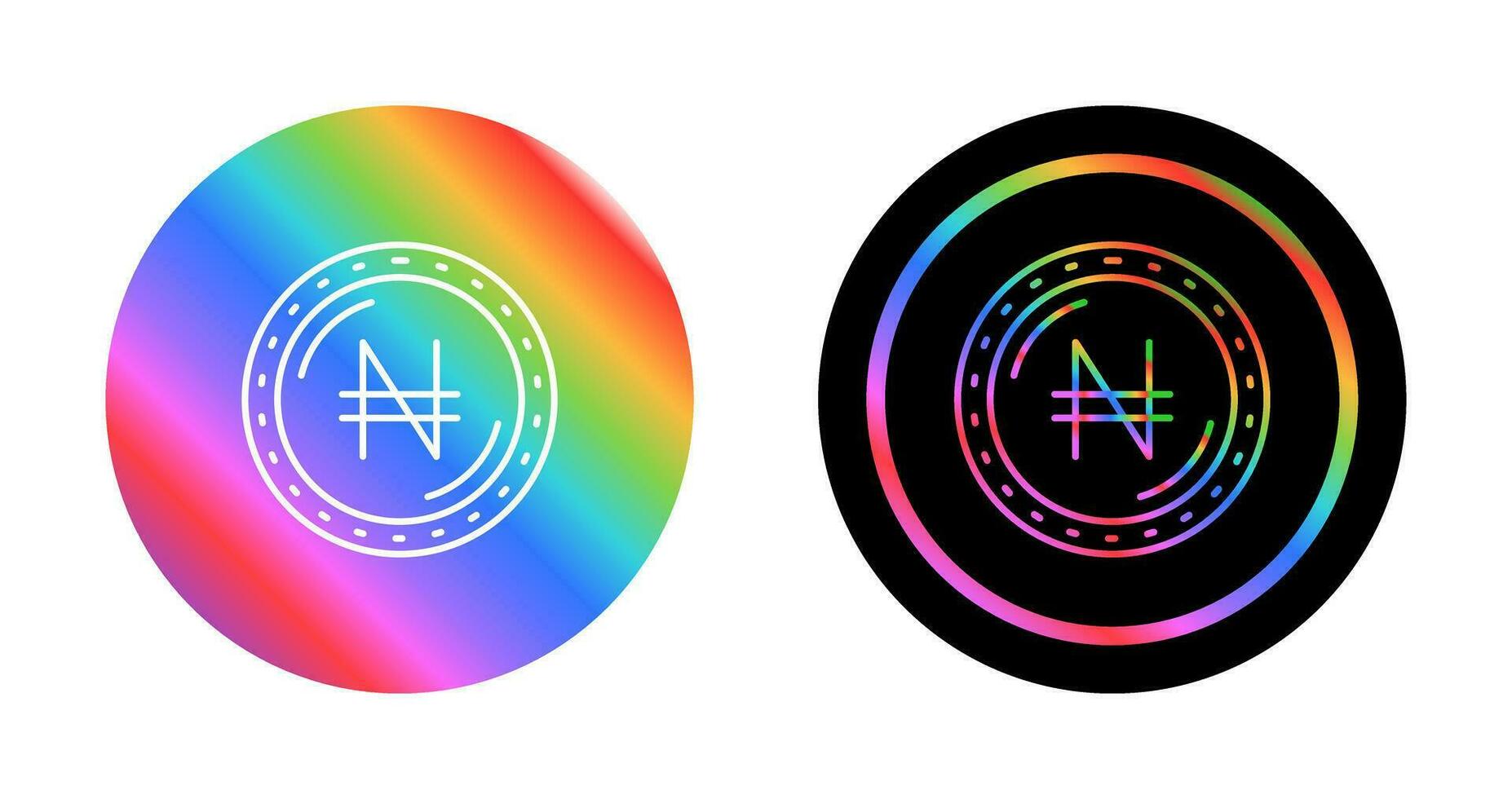This image features two circular, coin-like graphic designs placed side by side against a white background. Both designs prominently display the Naira sign (₦) in the center, with the symbol encased within a series of circular lines, mimicking a "circular road" motif. The left design showcases a vibrant, diagonal rainbow gradient that transitions from red at the top left, through a spectrum of colors, to red again at the bottom right. It contains a white circle with dotted and solid lines around the Naira symbol. The right design mirrors this structure but features a black background interspersed with rainbow-colored bars, maintaining the same circular, road-like element with the Naira symbol at its core. The overall composition highlights the contrast between the fully rainbow-colored left design and the predominantly black right design with rainbow accents.